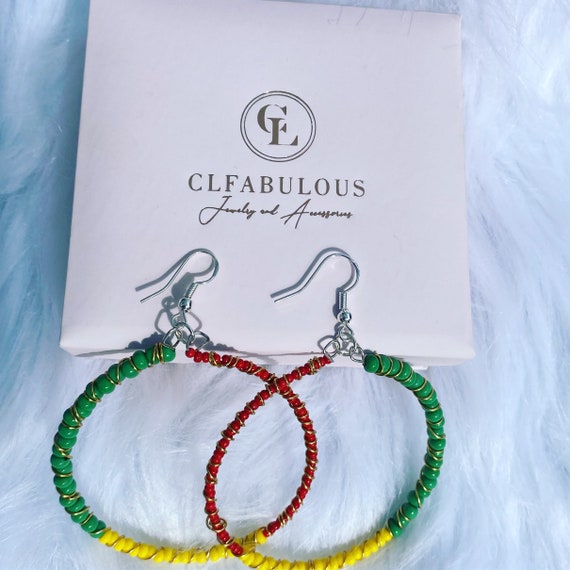This photograph features a pair of circular earrings, each divided into three sections of vibrant red, yellow, and green beads. The earrings are designed for pierced ears and are attached to silver metallic hooks. They rest on a small, square-shaped, white box or card. The box prominently displays a circular logo that reads "C.L." above the cursive brand name "C.L. Fabulous," which appears below the logo. The detailed accessories and the branding are set against a light blue fabric backdrop, suggesting they are carefully placed on a cloth for a studio-quality presentation.